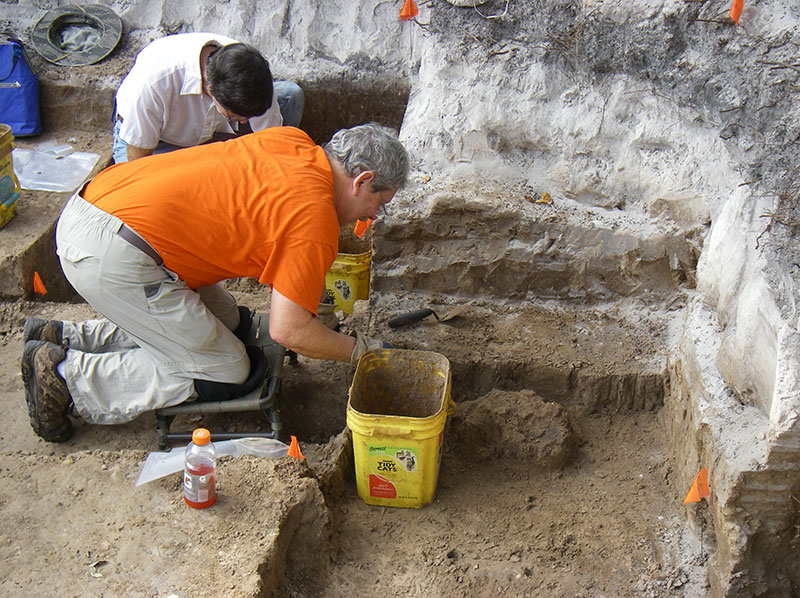The image depicts an archaeological dig site with two men meticulously working. The ground is stratified, showing layers of dark clay-like soil, a white band, and a top layer of pale gray rock, indicating possible volcanic activity. Central to the scene is an older man in a bright orange shirt, white pants, and brown shoes, with gray hair and glasses, hunched down on one of the excavated steps. A red Gatorade bottle is visible near him. Behind him, another individual, possibly younger and dressed in a white shirt, is also working on the site. Both men use yellow buckets to collect excavated material, and small flags mark specific points of interest around them. The steps they are uncovering appear to be formed from the same material filling their buckets. The surrounding environment adds to the sense of a cavern, with the gray rock walls transitioning from a darker shade at the top to a paler tone below.